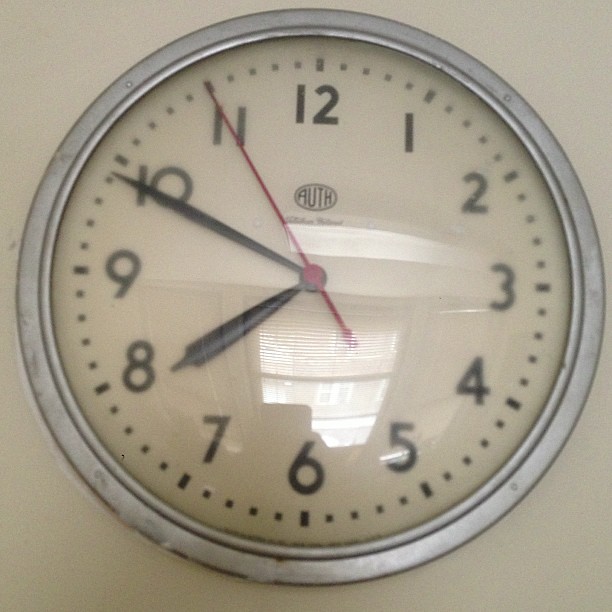The image depicts a classic wall clock set against a light to medium gray background, adding a somber, muted backdrop. The clock is encased in a medium gray metallic frame with visible patches of rust, hinting at age and wear. The clock’s face is a crisp white, providing a stark contrast to the bold black numerals marking the hours from 1 to 12. Each numeral sits within a vertically oriented rectangle, while smaller black squares mark the individual minutes between each numbered hour. The clock features three hands: a traditional black hour hand, a black minute hand, and a distinct red second hand. The time displayed on the clock is precisely 7:49.